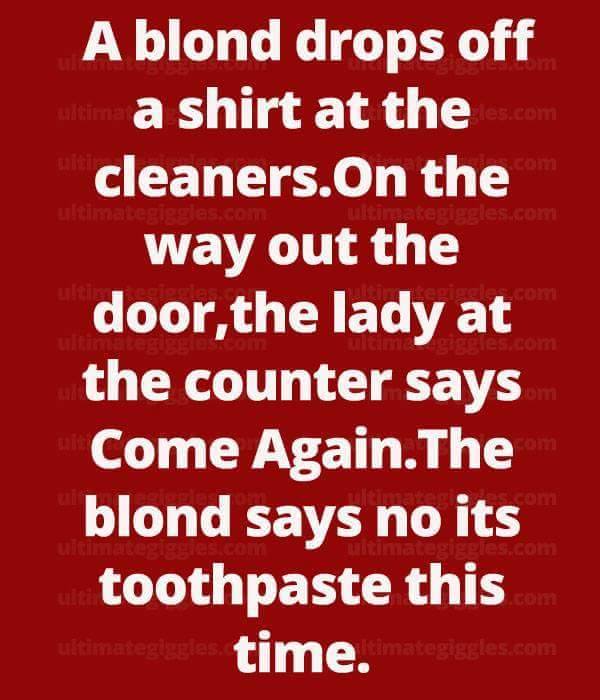Against a solid red background, this image features large, easily readable white text delivering a humorous joke: "A blonde drops off a shirt at the cleaners. On the way out the door, the lady at the counter says, 'Come again.' The blonde replies, 'No, it's toothpaste this time.'" Adding to the visual complexity, a faint watermark runs vertically on both sides of the image, consisting of two separate rows displaying "ultimategiggles.com." The watermark is barely discernible, blending seamlessly into the red background and requiring close inspection to read.